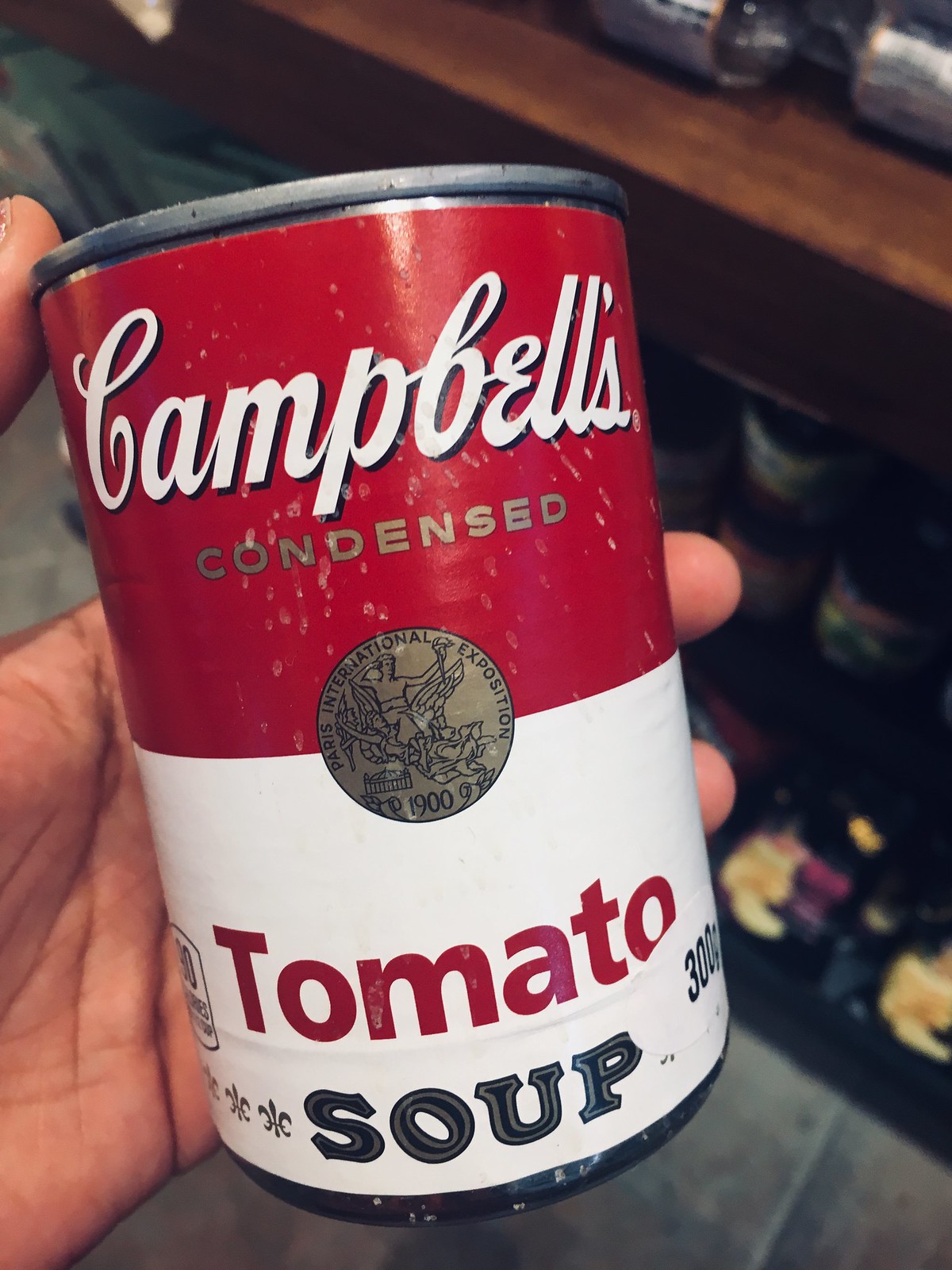The image captures a close-up of a hand on the left side of the frame, holding a can of Campbell's tomato soup. The hand's thumb and the tips of the forefinger and middle finger can be seen gripping the can. The classic Campbell's soup can, with its red and white label, appears weathered with a faded label and a few spots. The label features the iconic "CAMPBELL'S" in large cursive white letters on the red upper half, with "CONDENSED" in brown-gold capital letters underneath. At the center of the label is a round, bronze-colored circle with black details, likely depicting an emblem or figure. "TOMATO" is written in red lowercase letters just above the bottom white section, which reads "SOUP" in gray block letters, repeated with an inner outline in black. The background reveals a tile floor at the bottom and a wooden shelf, indicating a kitchen setting rather than a grocery store aisle.